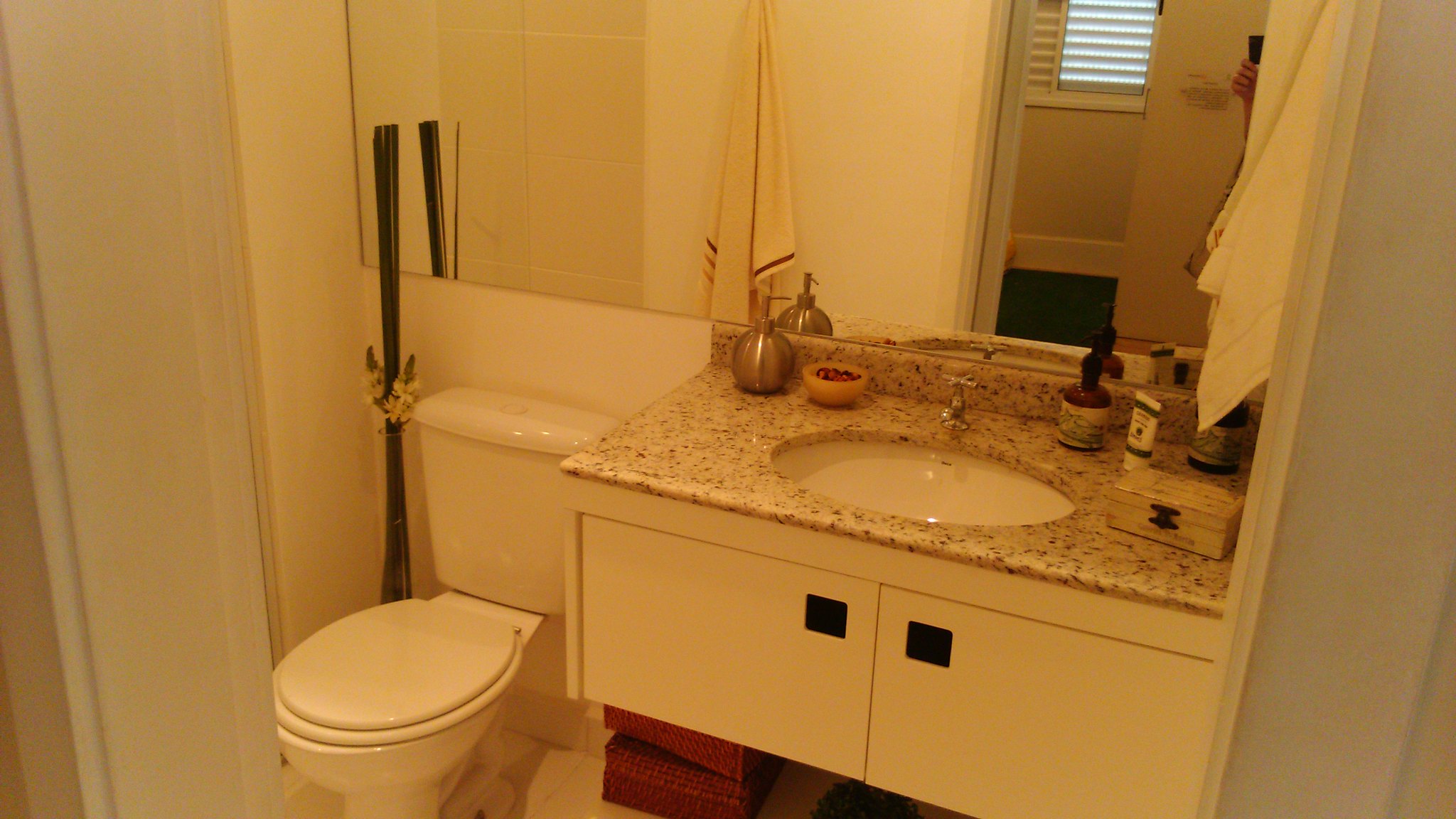This image showcases a meticulously designed bathroom within a house. To the left side of the frame, a pristine white toilet is positioned adjacent to an interesting arrangement of black rods or sticks, bound together by a decorative element resembling leaves, flowers, or ferns at the midpoint. 

Moving to the right, the sink area captures attention with its stylish marble countertop speckled with various shades of brown—light, dark, and even some reddish-brown accents. The sink itself is installed above a set of elegant white cabinets featuring distinctive black square handles. Situated discreetly beneath the sink, there are three small brown square objects that appear roughly the size of phone books, though their purpose remains unclear.

Occupying a place of prominence on the countertop, a sleek, metallic, spherical soap dispenser glistens in silver, while nearby, a tan bowl containing red spherical ornaments adds a touch of color and texture. The faucet, characterized by its singular turn knob, lacks conventional hot and cold controls. Further contributing to the counter’s theme of subdued elegance, there's a brown container with partially transparent sections and a light brown label accented with green. Alongside it stands a white cream bottle, embellished with green bands and illegible text, and finally, a brown box with a black latch.

On the right side of the bathroom, a crisp white towel is neatly hung. Complementing the space, a large wall-mounted mirror spans the entire area above the toilet and sink, reflecting part of the bathroom and a glimpse into an adjacent room. In the mirror’s reflection, one can spot a fragment of a person’s hand holding a phone, as well as the neighboring room characterized by a green floor, light brown walls adorned with white trim, and an open window fitted with blinds, partially revealing the outdoors.